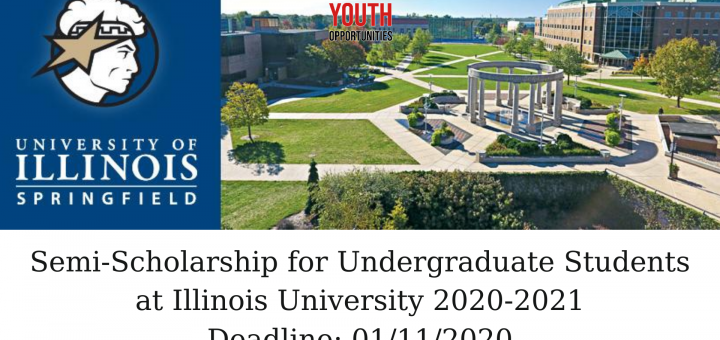This vibrant promotional image from an advertisement by the University of Illinois Springfield showcases the picturesque campus, highlighting the available youth opportunities. In the middle of the frame, the text "Youth Opportunities" stands clear and prominent. The campus scene features numerous elegant buildings, lush green lawns, and mature trees, all connected by neat sidewalks. Centrally located is a distinctive circular gazebo-like structure with open walkways supported by pillars.

On the left side of the image, a blue rectangular banner features a cartoonish gladiator figure with a star emblem, rendered in tan. Against the blue background, the university's name is displayed: "University of Illinois" with "Springfield" separated by a line beneath it. The promotional text emphasizes "Youth" in bold red letters, followed by additional details in black.

Below, it reads: "Semi-Scholarship for Undergraduate Students at Illinois University 2020-2021," with a crucial note on the application deadline: "01/11/2020," though partly obscured. This compelling visual advertisement aims to attract prospective students by highlighting both academic opportunities and the scenic campus environment.